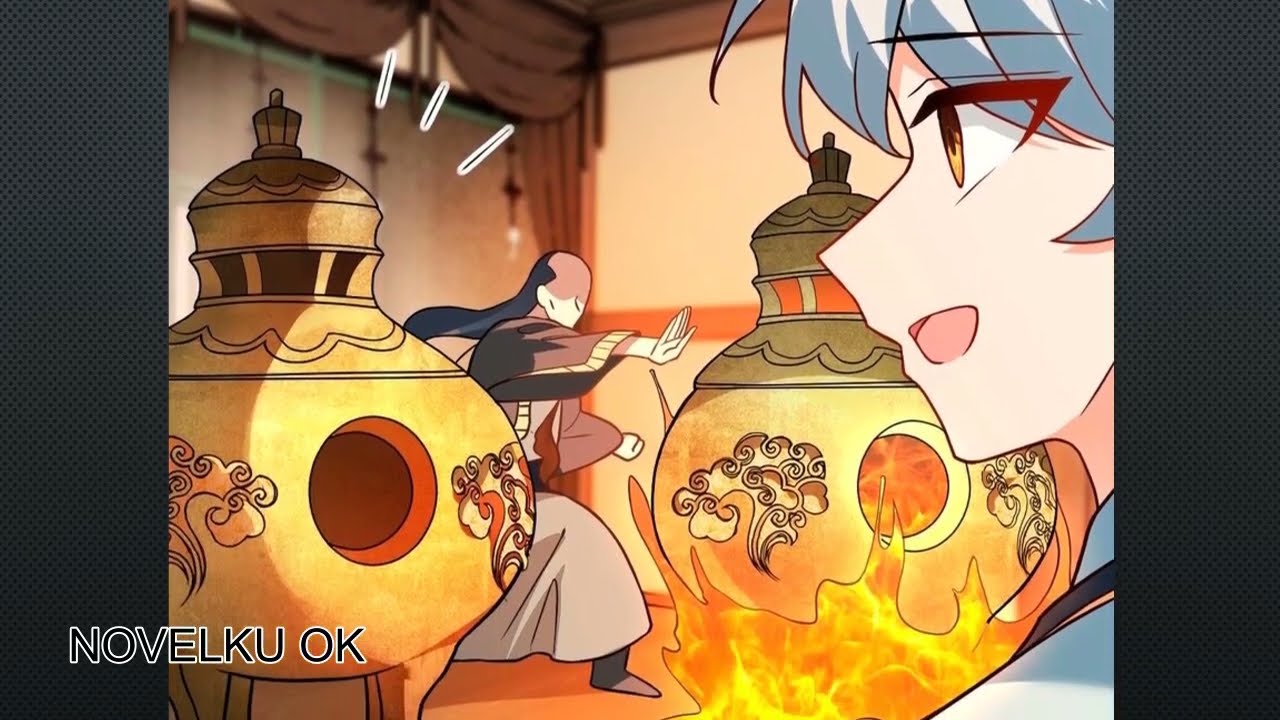The image is a detailed panel from a webcomic, bordered vertically by dark gray bars featuring a honeycomb pattern. The bottom left corner displays the text "NOVELKU OK" in black font with a white outline. The central scene appears to be set inside a traditional Japanese building, reminiscent of anime or manga style. 

On the right side of the panel, a character with pale skin, silver-blue hair, and light blue eyes is depicted with an open mouth as if speaking. He is wearing a light blue shirt and smiling at an empty vase next to a large clay pot. 

To the left, another character with light skin and a receding hairline has long black hair. He is dressed in traditional Japanese robes and is striking a martial arts pose toward another giant clay pot, which is emitting flames from its base and interior. The setting and elements such as the traditional Japanese clothing and pots reinforce the cultural ambiance of the scene.